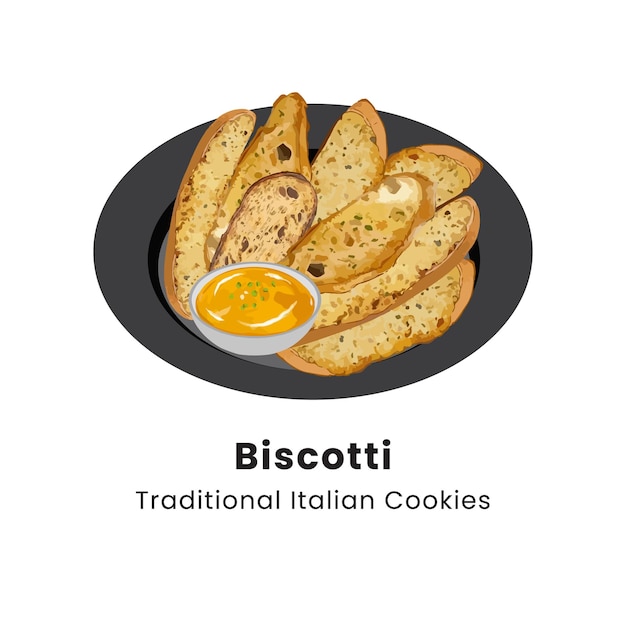This image, resembling a well-executed painting or drawing, features a dark gray plate set against a stark white background. On the plate lies an assortment of long, beige, cream, and brown biscotti—Italian cookies baked until dried, traditionally meant to be enjoyed with coffee. The biscottis appear fresh yet characteristically dry, speckled with small brown and green dots. There are eight pieces in total, arranged around a small, white bowl filled with a yellow-orange dip, adding an unusual twist to the traditional coffee accompaniment. Black lettering at the bottom of the image reads, "biscotti, traditional Italian cookies," adding an informative touch to the artistic representation.